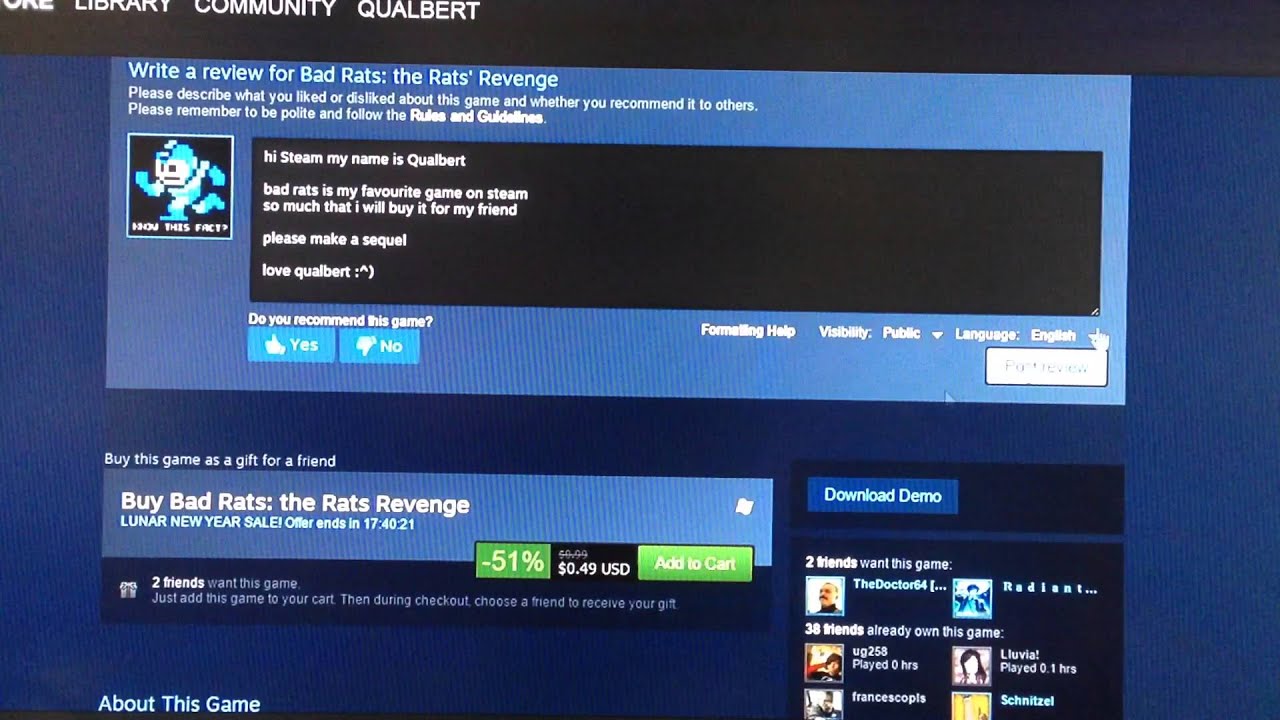**Descriptive Caption:**

The image is a screenshot from a digital interface, possibly from a mobile app or gaming console. The interface features a dark-themed header with white text displaying the sections: "Library," "Community," and the username "Qualbert." Below this, a light blue section prompts the user to write a review for the game "Bad Rats: The Rats' Revenge." It encourages the user to share their likes, dislikes, and recommendations while reminding them to adhere to guidelines and be polite.

Embedded in this section is an avatar of Classic Mega Man with the text "How this fact" or "Now this fact?" followed by a user review by "Qualbert." The review reads: "Hi, Steam. My name is Qualbert. Bad Rats is my favorite game on Steam, so much that I will buy it for a friend. Please make a sequel, love, Qualbert," punctuated with a sideways smiling emoji.

Below the review, the user is asked if they recommend the game, with light blue buttons for "Yes" (thumbs up) and "No" (thumbs down). To the right, options for "Formatting help" and a visibility setting (public) with a language dropdown (English) are available.

Further down, there's an option to buy the game as a gift for a friend during a Lunar New Year sale, which ends in "17:40:21" (a countdown timer). The sale price is prominently displayed as "$0.49" (down 51% from the original price, which is crossed out but difficult to read). Next to it, a green "Add to Cart" button is clearly visible. Additionally, there is a "Download Demo" button, offering users a chance to try the game before making a purchase.